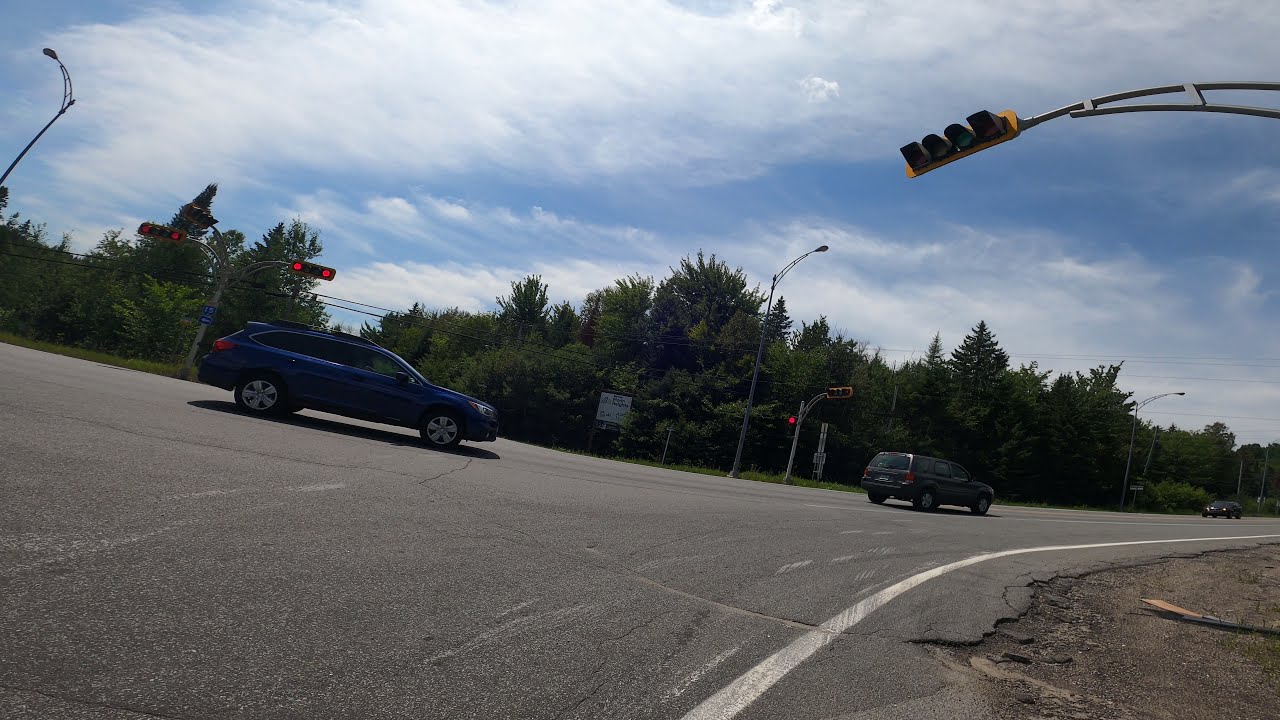The image is a high-quality, horizontally aligned photograph taken outdoors at ground level, capturing a road intersection. The top portion displays a bright blue sky with delicate, feathery white clouds. In the middle background, a densely forested area showcases tall green trees, including some evergreens and deciduous trees with fluffy crowns. 

Two cars are traveling from left to right on this wide, gray roadway. The first, a gray SUV, is followed closely by a royal blue Subaru-like station wagon. From the opposite direction on the far right side, a sporty car resembling a Corvette approaches these two vehicles. Traffic lights, distinctly showing red, are positioned to the left of the blue station wagon, with another traffic light visible but without discernible signals in the upper right corner. The road also features a solid white stripe marking the shoulder. The scene is naturally lit, with bright and clear lighting, making all the details easily visible.